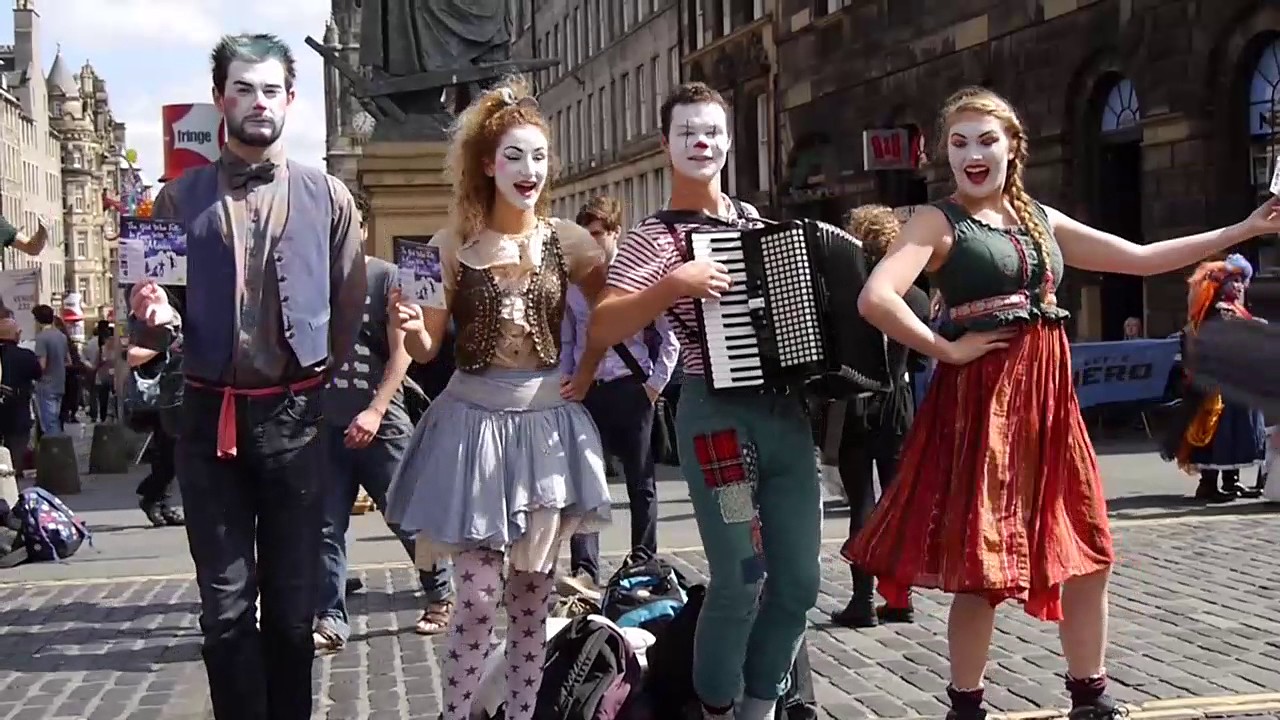In this lively street scene, four pantomime performers stand in a row on a gray cobblestone courtyard, framed by a bustling cityscape and onlookers. Each has their face painted white, accented by vivid makeup. On the far left, a man with green hair wears a blue vest, red belt, and black pants, showcasing a card in his right hand. Next to him stands a blonde woman with her hair up, dressed in a gold top, gray vest, blue skirt, and star-patterned pink leggings. The third performer, a man with a striped red shirt, green patched pants, and a red nose, joyfully plays an accordion. On the far right, a smiling blonde woman, sporting pigtails, wears a black tank top and a vibrant skirt, her right hand poised on her hip and her left arm outstretched. The cobblestone street beneath them is lively with city activity, providing a dynamic backdrop to their captivating performance.